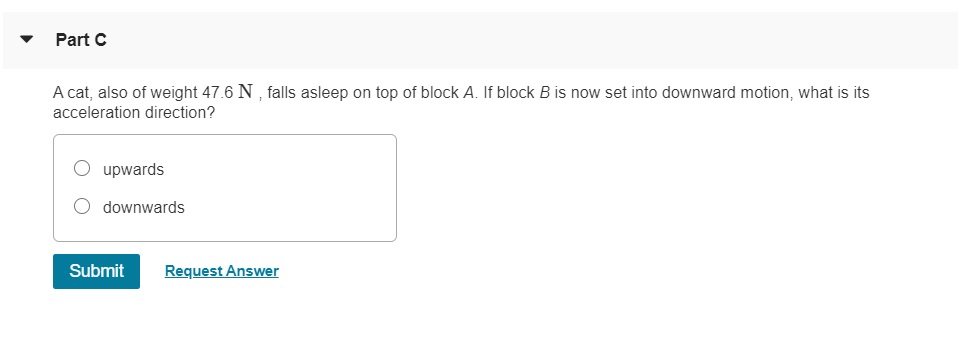This is a detailed descriptive caption for the screenshot:

The image depicts a screenshot of a computer screen displaying a section from an educational interface. The interface features black text on a white background, with a distinct gray rectangular bar spanning the top of the screen. In the upper left of this bar, bold black text reads "Part C," accompanied by a small downward-pointing triangle. Below this gray bar, there is light gray text providing a problem statement: "A cat, also of weight, 47.6 N, falls asleep on top of block A. If block B is now set into downward motion, what is its acceleration direction?"

Following the problem statement, there is a horizontal gray rectangle that serves as a placeholder for multiple-choice options. Next to this rectangle, there are two clickable circles (radio buttons). The first circle is labeled "upwards," and the second circle is labeled "downwards."

At the lower left corner of the screen, a turquoise blue rectangle labeled "Submit" offers an option to submit an answer. To its right, in the same turquoise color and underlined, is the text "Request Answer," providing an option to reveal the correct answer upon clicking.

This educational interface seems to be designed for interactive learning, where students can select and submit their answers or request the correct answer for immediate feedback.